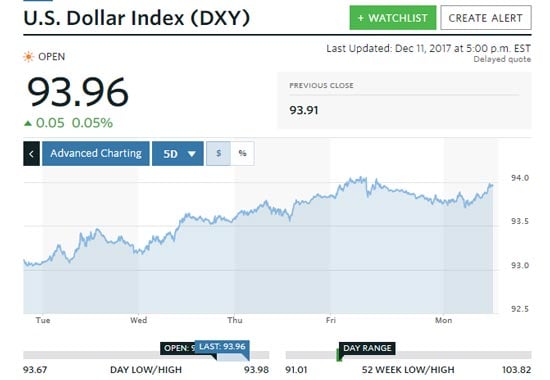The image depicts a comprehensive stock chart for the U.S. Dollar Index (DXY). The index is prominently displayed at the top, with an arrow indicating a rising trend towards the right. Adjacent to this, there is a green button labeled "+ Watch List" in white text, indicating an option to add the index to a watch list. Beside it, a white button labeled "Create Alert" in gray text offers the functionality to set an alert for the index.

Below the title, a horizontal underline stretches from left to right, extending under the "U.S. Dollar Index", "Create Alert", and "+ Watch List" sections. Underneath this underline, there is a sun symbol followed by the word "OPEN" in capital letters. The last update is recorded as December 11, 2017, at 5 p.m. Eastern Standard Time, with a note that the quote is delayed.

The current quote is displayed as $93.96, an increase of $0.05 or 0.05%. To the right, another box labeled "Previous Close" shows the previous closing value of $93.91 with a light gray line highlighting this section.

The lower section showcases the actual stock chart, accompanied by options such as "Advanced Charting". Below the chart, a five-day outlook is provided, listing the days of the week: Tuesday, Wednesday, Thursday, Friday, and Monday.